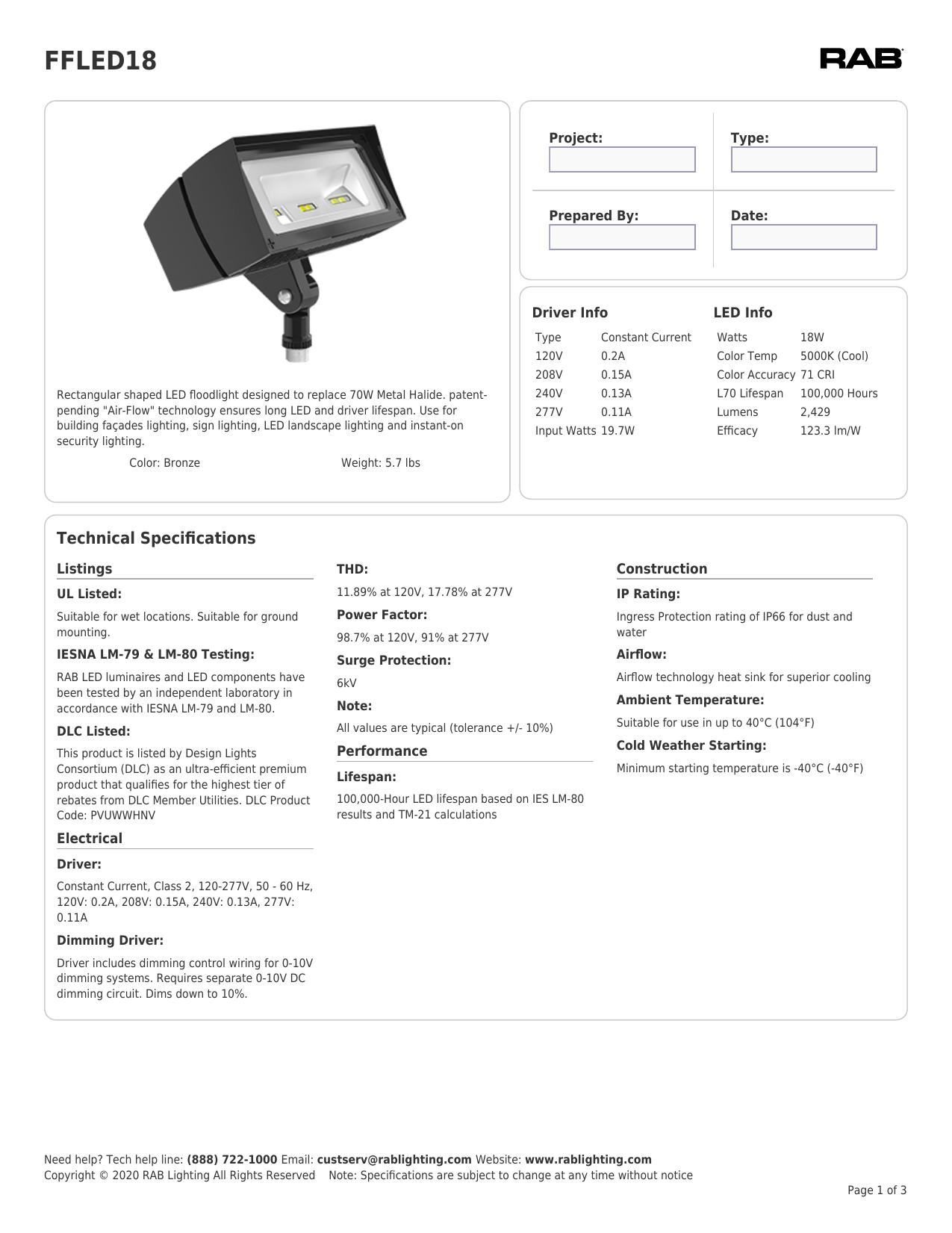**Detailed Caption:**

The image displays a well-organized and informative page featuring product details and technical specifications for a specific light fixture. At the top of the page, the model number "FFLED18" is prominently displayed, and the brand "RAB" is noted in the top-right corner.

**Section 1:**
Located in the top-left, this section includes an image of the light fixture, which is black in color. The descriptive text reads: "Rectangular-shaped LED flat light designed to replace 70W metal halide, patent pending. Airflow technology ensures a long LED and driver lifespan. Suitable for building side lighting, landscape lighting, and instant-on security lighting." Additional details include its bronze color and weight of 5.7 lbs.

**Section 2:**
Positioned in the top-right, this section includes a form with fields for "Prepared by," "Type," and "Date," allowing users to fill in relevant details as needed.

**Section 3:**
Below the form, on the right, is a section titled "Driver Info and LED Info." It provides technical specifics such as the type being "constant current," a power consumption of 18 watts, and multiple input voltages (12V, 228V, 240V, 277V).

**Section 4:**
At the bottom of the page is the "Technical Specifications" section, detailing various aspects including listing, electrical characteristics, dimming capabilities, driver type, construction materials, IP rating, airflow properties, suitable ambient temperature ranges, cold-weather operation, lifespan, surge protection, and power factor.

The footer of the page indicates it is "Page 1 of 3" and provides contact information: a helpline number (888-722-1000), an email address (castself@replighting.com), and the company website (www.replighting.com).